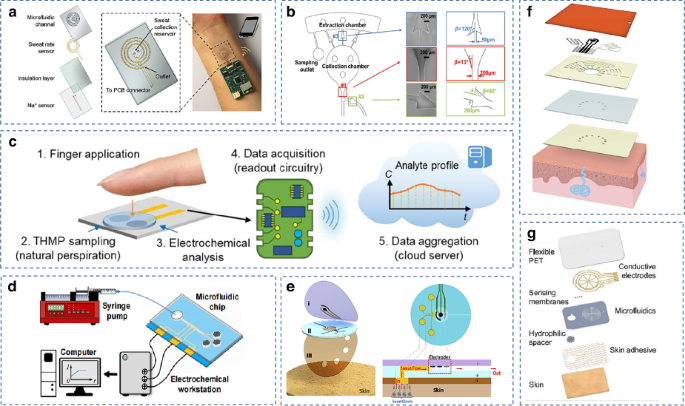This detailed and colorful diagram illustrates a complex medical process involving a microfluidic device designed to sample and analyze perspiration directly from the finger. The poster, sectioned into seven distinctive parts labeled A through G, meticulously presents each step of the process. It begins by instructing on how to correctly place a finger on the small circuit board equipped with conductive electrodes and skin adhesive. Subsequent panels detail the internal components and functionality of the device, including elements like data acquisition and aggregation mechanisms integral to the microfluidic chip. Arrows and extensive black text annotations guide the viewer through each stage, making the intricate procedure accessible to those with a technical background. The vibrantly colored sections and clear breakdown of steps highlight the innovative method for real-time sweat analysis and precise data upload, underscoring the practical interaction between biological data and microelectronic technology.